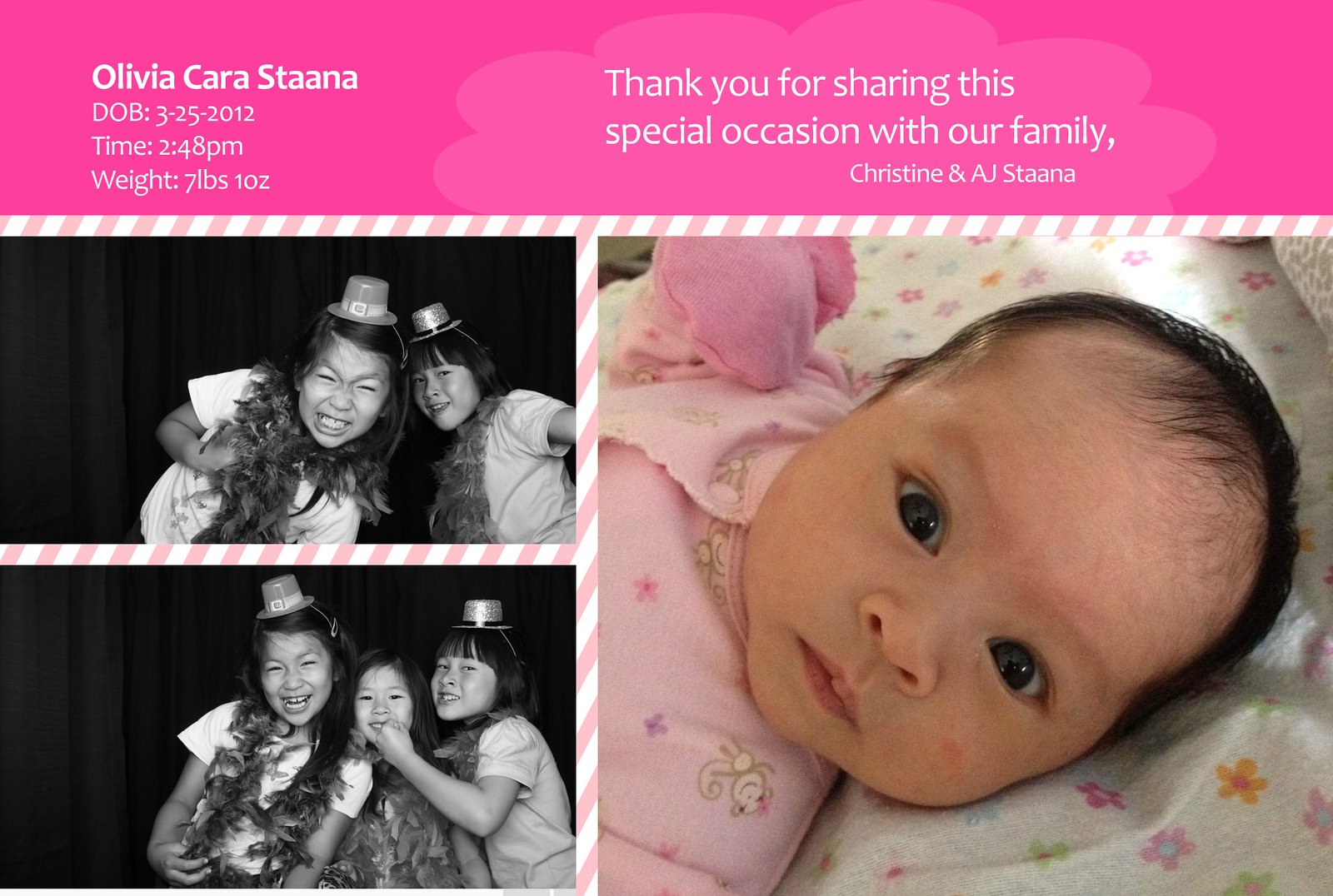This is a baby announcement for Olivia Kera Stanna. The top 20% of the announcement features a bright pink banner with white text that reads: "Olivia Kera Stanna, Date of Birth: 3-25-2012, Time: 2:48 p.m., Weight: 7 lbs 10 oz." Below this is a lighter pink flower-like outline containing the message, "Thank you for sharing this special occasion with our family, Christine and A.G. Stanna."

The bottom two-thirds of the announcement is divided into sections. On the right, there's a color photograph of baby Olivia, who has dark brown (almost black) hair, blue eyes, and is wearing a pink shirt with matching mittens to prevent her from scratching her face. She is pictured looking up at the camera from her baby bed.

To the left, there are two black-and-white photos. The upper photo shows two girls, around 8 to 10 years old, possibly of Asian descent, wearing T-shirts, hats (resembling St. Patrick's Day hats), and Hawaiian leis. They are looking intensely at the camera, with one girl smiling broadly and the other with a smaller smile. The lower photo features these same two girls with an additional girl positioned between them. All three are laughing and appearing to have more fun compared to the upper image, still wearing their festive costumes. The announcement captures a joyous and intimate family moment, celebrating the arrival of baby Olivia amidst her loving family.